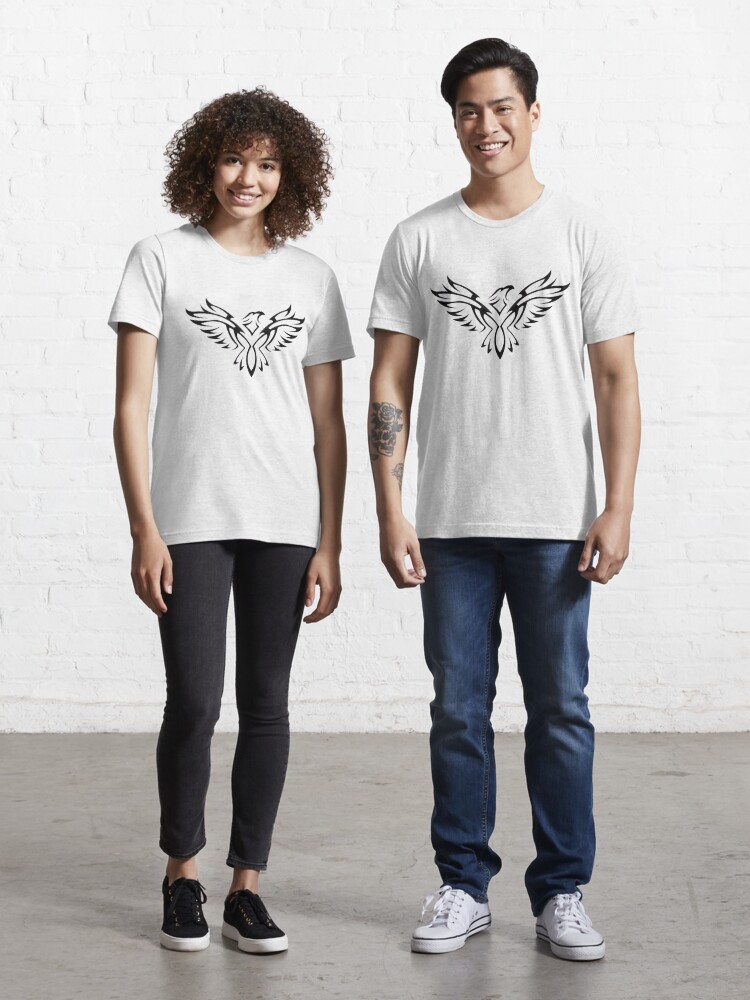The image features a promotional photo likely from a print-on-demand t-shirt company, showcasing a man and a woman standing side by side in matching white t-shirts. These t-shirts have a black stencil design of a phoenix rising from the ashes, depicted in a tribal style. Both models are smiling and staring directly at the camera, standing against a white brick wall on a gray cement floor. The man, who appears to be of Asian descent, is taller, wearing neat blue jeans and white canvas shoes, and has a tattoo of a skull with a flower on his right arm. He has thick, slicked-back black hair. The woman, possibly of Hispanic or African American descent, has shoulder-length ringlet curly hair. She is dressed in slim-cut black jeans and black canvas shoes with white soles. They both exude a casual yet coordinated look, perfectly fitting the clean and simple backdrop.